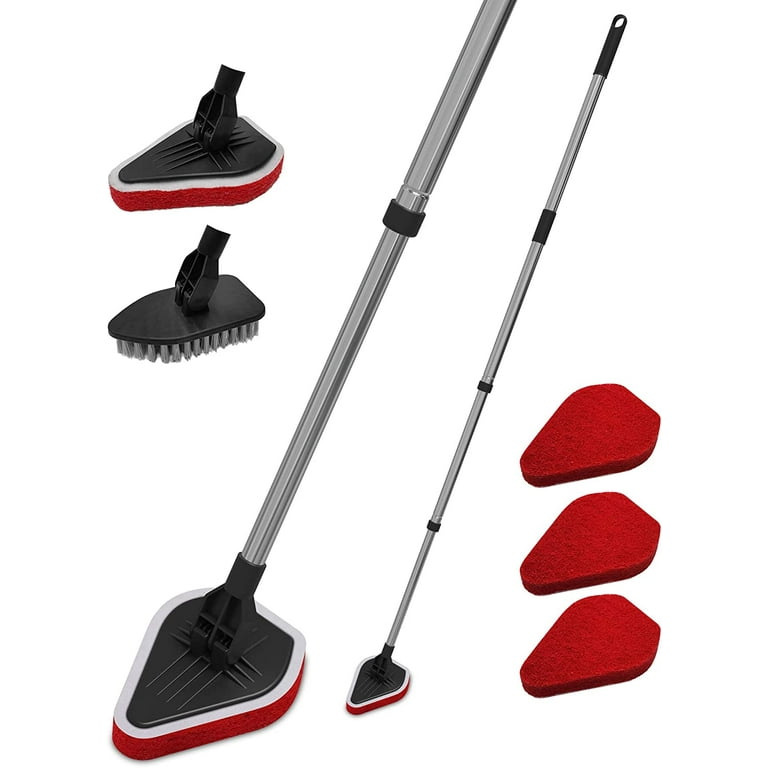The image shows an adjustable, long-handled telescoping cleaning device designed for versatile use on floors, walls, and potentially cars. The cleaning tool features a silver handle that can expand or collapse like a tripod leg, allowing for variations in length to suit different cleaning needs and user heights. The triangular base of the implement serves as the cleaning attachment point, where two different heads can be affixed: a red fabric cleaner and a brush with gray bristles. The red fabric cleaner head is sponge-like and attaches via a black connector, while the multi-functional brush provides more scrubbing power. Additionally, three replacement red fabric sponges are displayed to the right of the image, indicating the availability of refill options. The images include different views such as a full-length shot of the device, a close-up of the telescoping mechanism, and individual shots of the interchangeable cleaning heads. The white background emphasizes the details and components of this all-in-one cleaning tool, making it clear and easy to identify its various parts and functionality.